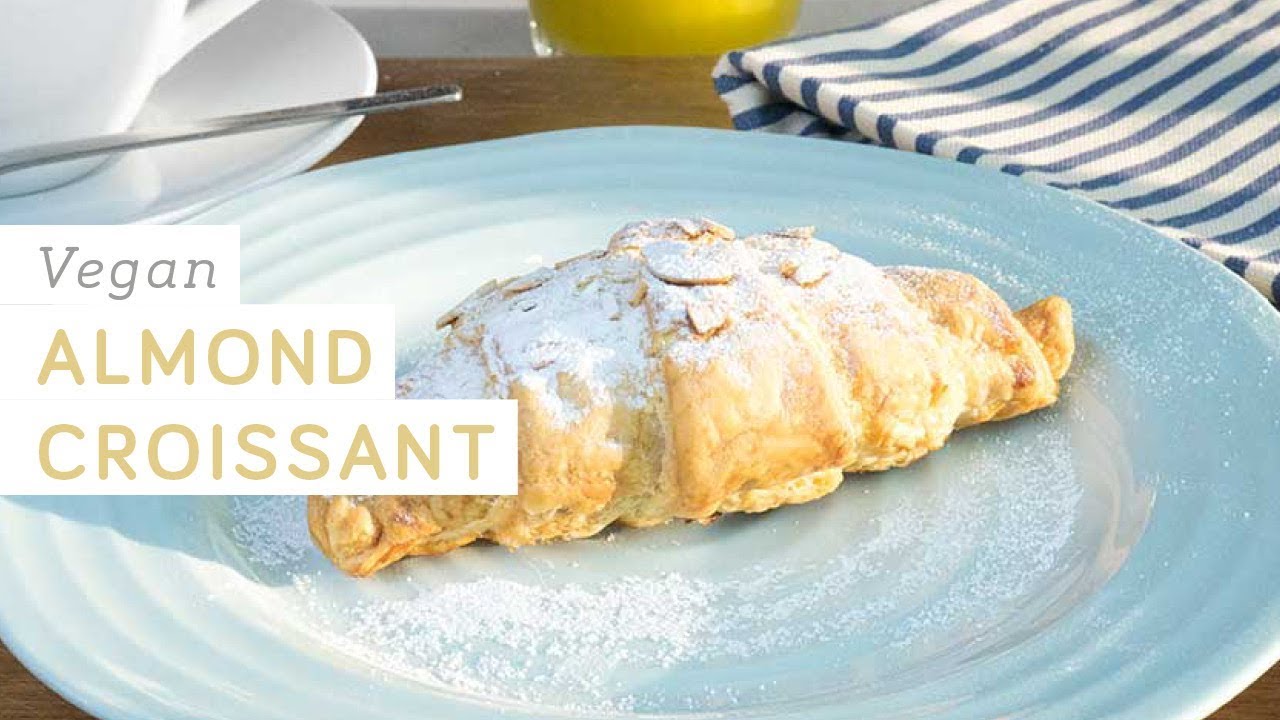The image depicts a neatly arranged, inviting scene centered around a vegan almond croissant on a light blue plate. The croissant, characterized by its orange and yellow tones, is generously topped with slivers of almonds and a dusting of powdered sugar, which also adorns the plate. On the left upper side of the image, a white teacup with a saucer and spoon is partially visible, adding a touch of elegance to the setting. Directly above the croissant, a hint of an orange juice glass peeks into the frame. A folded cloth napkin with alternating dark blue and white stripes lies to the right of the plate. Above the scene, a white rectangle with gray and light brown font prominently declares "Vegan Almond Croissant." All the elements rest atop a dark wood table, providing a rich, contrasting background that highlights the vivid colors and textures of the items.